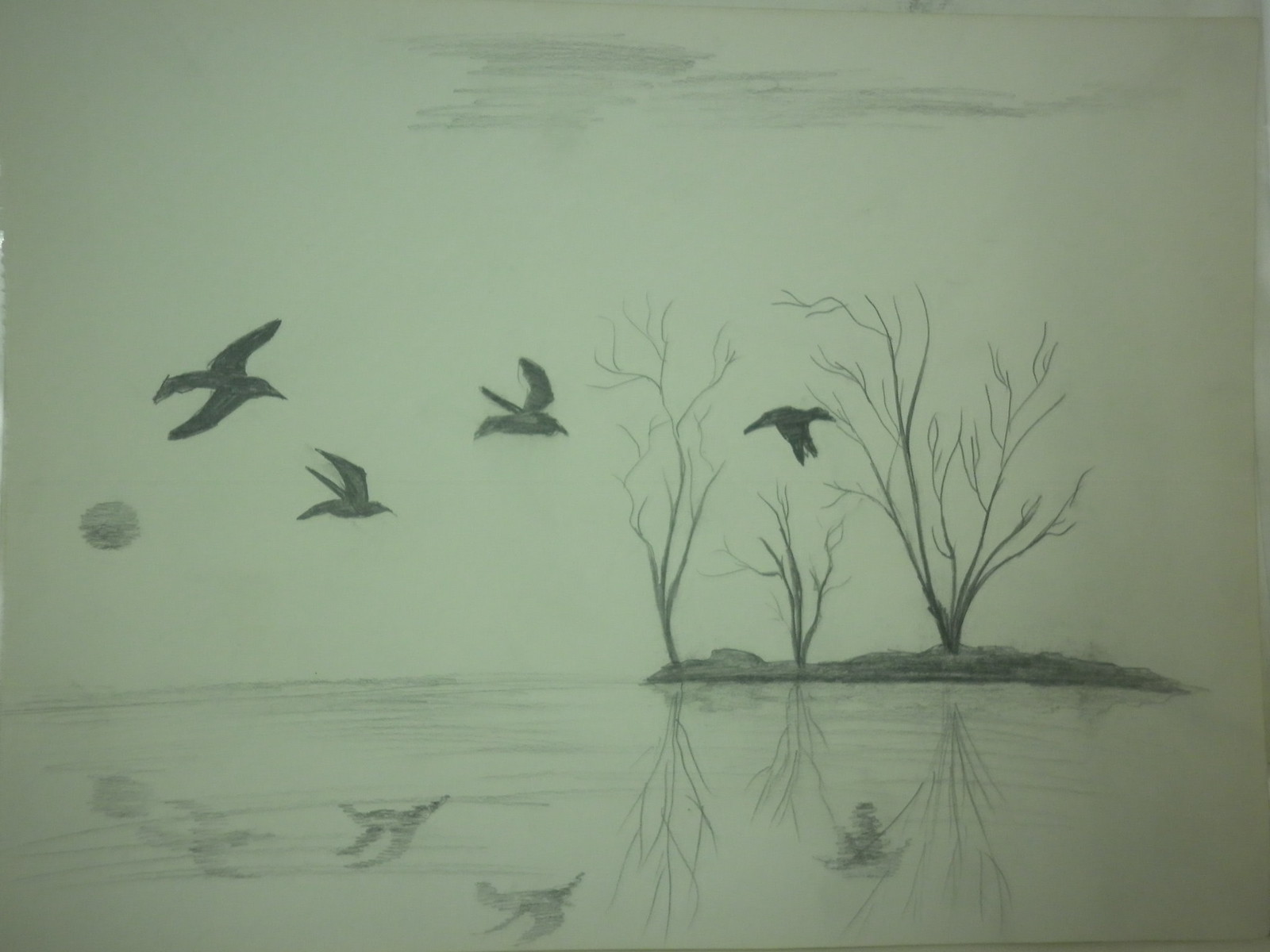The image is a hand-drawn, black-and-white illustration on greenish-colored paper, appearing to have been scanned into a computer. It depicts a serene water scene with four birds flying across the central area of the composition. Each bird is captured mid-flight with wings in varying positions, one even extending straight down towards the water. The water beneath them reflects their silhouettes, emphasizing the reflective surface.

In the background, on the right, there's a small island with three barren trees, their trunks and branches starkly outlined without any leaves. The top portion of the illustration features lightly sketched clouds created with gentle pencil strokes, adding to the drawing’s subtle atmosphere. To the left of the birds, a shaded circular object, possibly representing the sun or the moon, hovers above the water, contributing to the overall tranquility of the scene.